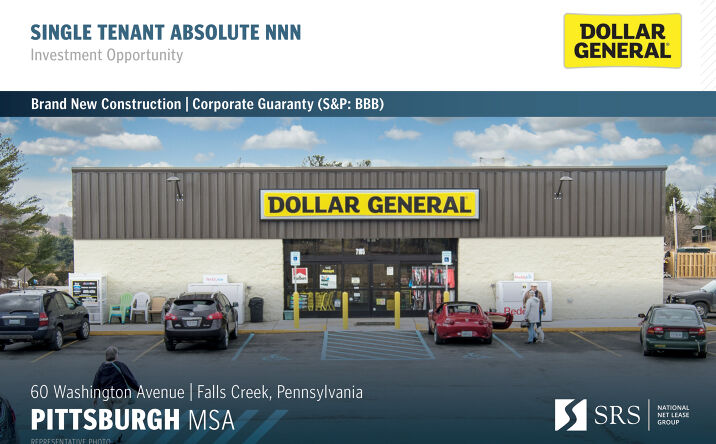This detailed advertisement image depicts a brand-new construction Dollar General store located at 60 Washington Avenue in Falls Creek, Pennsylvania, part of the Pittsburgh MSA. The S&P BBB-rated store boasts a prominent yellow and black Dollar General sign atop a brown awning. The building itself is cream-colored, with four handicap parking spots in front. The parking lot features several cars, including a red car, two black cars, and a green car. 

Notably, there are three people walking towards the store, and an ice chest for purchasing ice sits outside. Additionally, an unusual sight is the Marlboro cigarette sign near the entrance. The exterior setting includes a green, white, and beige area and possibly small propane gas containers. The image emphasizes the SRS company's involvement and highlights the single tenant absolute NNN corporate guarantee, ensuring a solid investment.